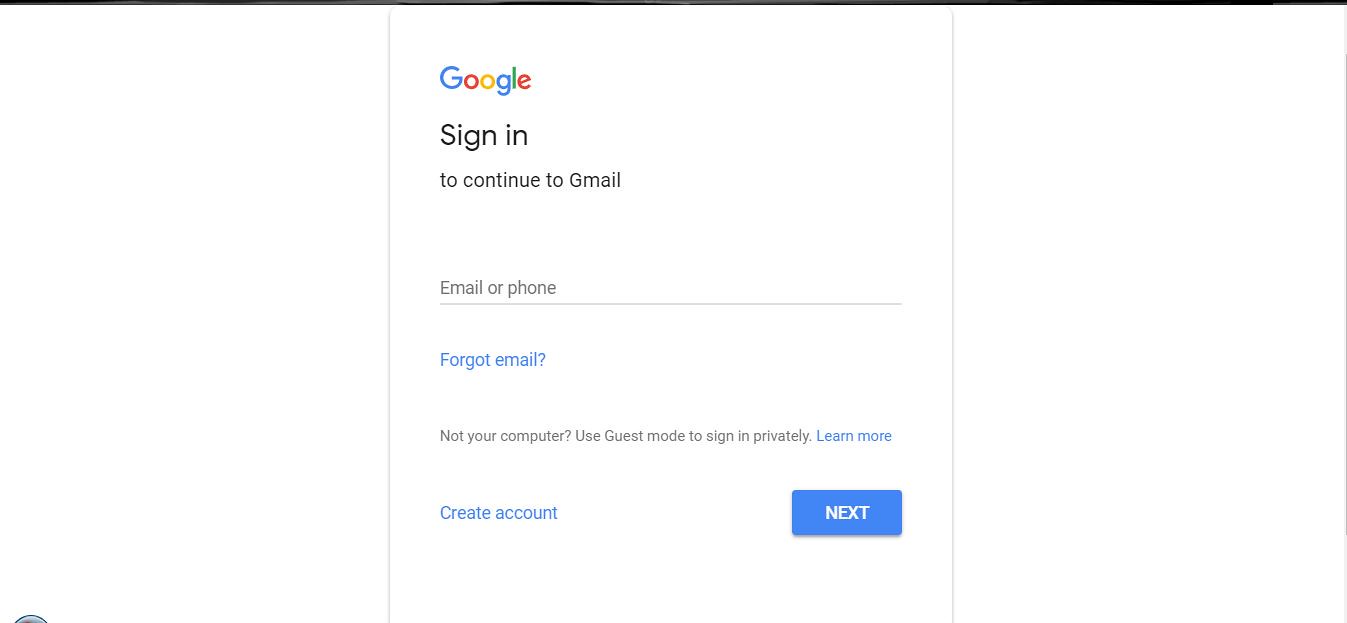This color photograph appears to be a screenshot of a Google sign-in page displayed on a computer screen. The background is predominantly white, ensuring a clean and straightforward presentation. At the top center of the image is the iconic multicolored Google logo, with each letter in "Google" in its signature colors: blue, red, yellow, blue again, green, and red.

Below the logo, the text prompts the user to "Sign in to continue to Gmail." It includes a field where users can enter their email or phone number, accompanied by a clickable "Forgot email?" link for those who need help recalling their login details.

Further down, an advisory message reads, "Not your computer? Use Guest mode to sign in privately," which directs users to learn more via a hyperlink. Underneath, another link invites users to "Create account" if they don't already have one.

The main interactive element is a prominent blue "Next" button, which users press after entering their information to proceed with the sign-in process. Most text on the page is rendered in black, maintaining a clear and professional appearance, while hyperlinks and action buttons are highlighted in blue for easy navigation. The visual hierarchy and color scheme are in line with Google's trademark minimalistic and user-friendly design ethos.